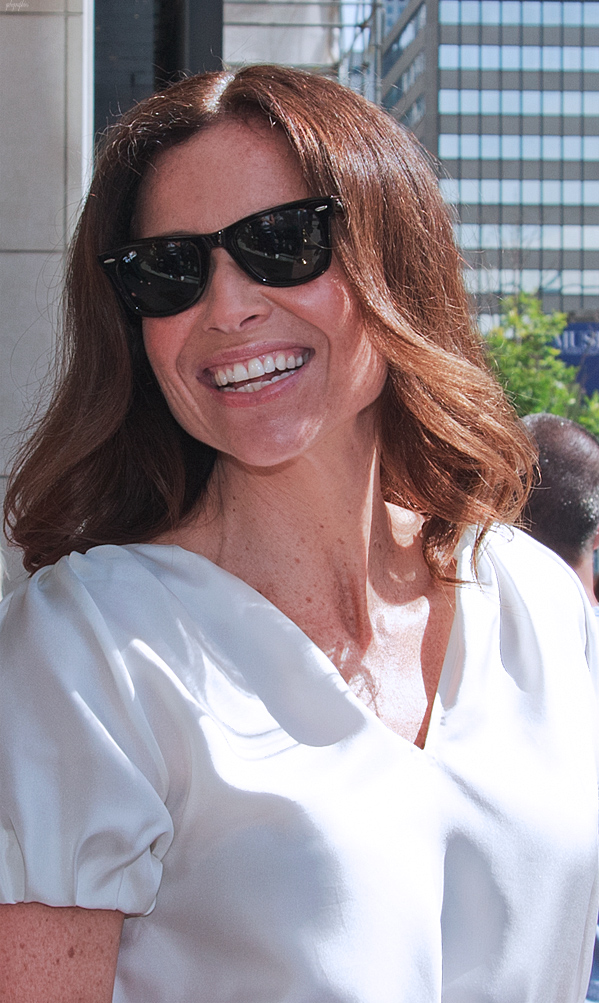The photo features actress Minnie Driver, appearing to be in her late 40s to early 50s. She is outdoors, with buildings and high rises in the background, as well as what appears to be another person to her right. Minnie is wearing black sunglasses that obscure her eyes but is smiling broadly, exuding happiness. Her light brown, slightly wavy hair cascades just past her shoulders with a bit of a curl at the bottom. She is dressed in a white blouse, which appears to be made of silk, and it has short sleeves that don't quite reach her elbows. The blouse has a V-neck, revealing a few moles and freckles on her neck and arms. Overall, the image captures her joyous demeanor and the lively urban environment around her.